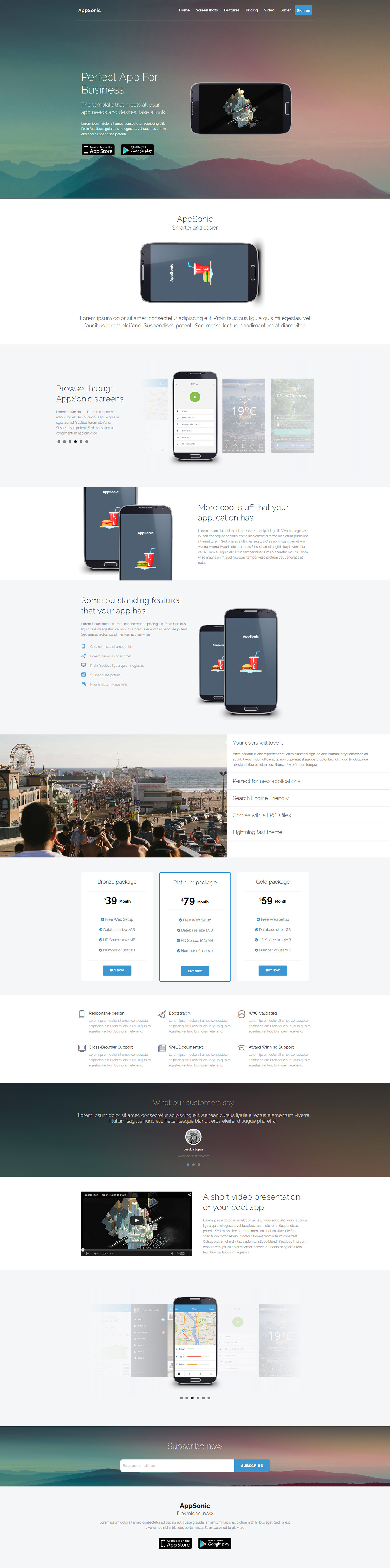**Detailed Website Screenshot Description:**

The screenshot captures the entire length of a website, presented in a condensed, vertical format that eliminates the need for scrolling. At the top of the page, a scenic header image featuring mountaintops or hills is overlaid with a striking blue, orange, and yellow gradient. Above this image, a small, white navigation menu is barely discernible due to its size.

Centered within this header image, the white text announces "Perfect App for Business," accompanied by secondary white text below it. Two prominently displayed buttons invite users to download the app from the Google Play Store or the Apple App Store. Adjacent to this text, a horizontally-oriented black smartphone displays a graphic or image.

Directly beneath the header, a white panel houses another horizontally-oriented smartphone. The screen shows an image of a hamburger and a Coke soft drink against a gray background. Small black text is positioned above and below this image, providing additional context.

Following this section is a light gray panel featuring a mobile device with screenshots of three different screens displayed next to it. Below this, another thin, white rectangular panel showcases images of two mobile phones, both displaying the same hamburger and Coke image, with small adjacent text.

A subsequent light gray rectangular panel is positioned to the left, containing descriptive writing to the right and two wider tablet devices beneath this text. Each tablet displays the dark gray background and the same hamburger and drink image in the center.

Next, a panel features an outdoor scene with a crowd of people, a distant Ferris wheel, and a body of water. To the right of this vibrant image, a white information panel provides further details.

Descending further, a light gray panel on the left presents text, while the right side displays three square segments with different pricing options. Each pricing box includes a price, bullet points, and a blue button.

This is followed by a white square panel with grayish-black text. Below this, a greenish-grayish-orange panel contains white text.

Further down, another white rectangular panel shows a long screen resembling a monitor or TV, accompanied by text on the right.

The next section includes a gray block with a tablet device displaying a navigation screen. A small, thin block with a green, brown, and orange gradient houses a text box and a blue button.

Finally, the bottom part of the website concludes with a light gray section containing text and two more buttons for finding the app in the iStore and the Google Play Store.